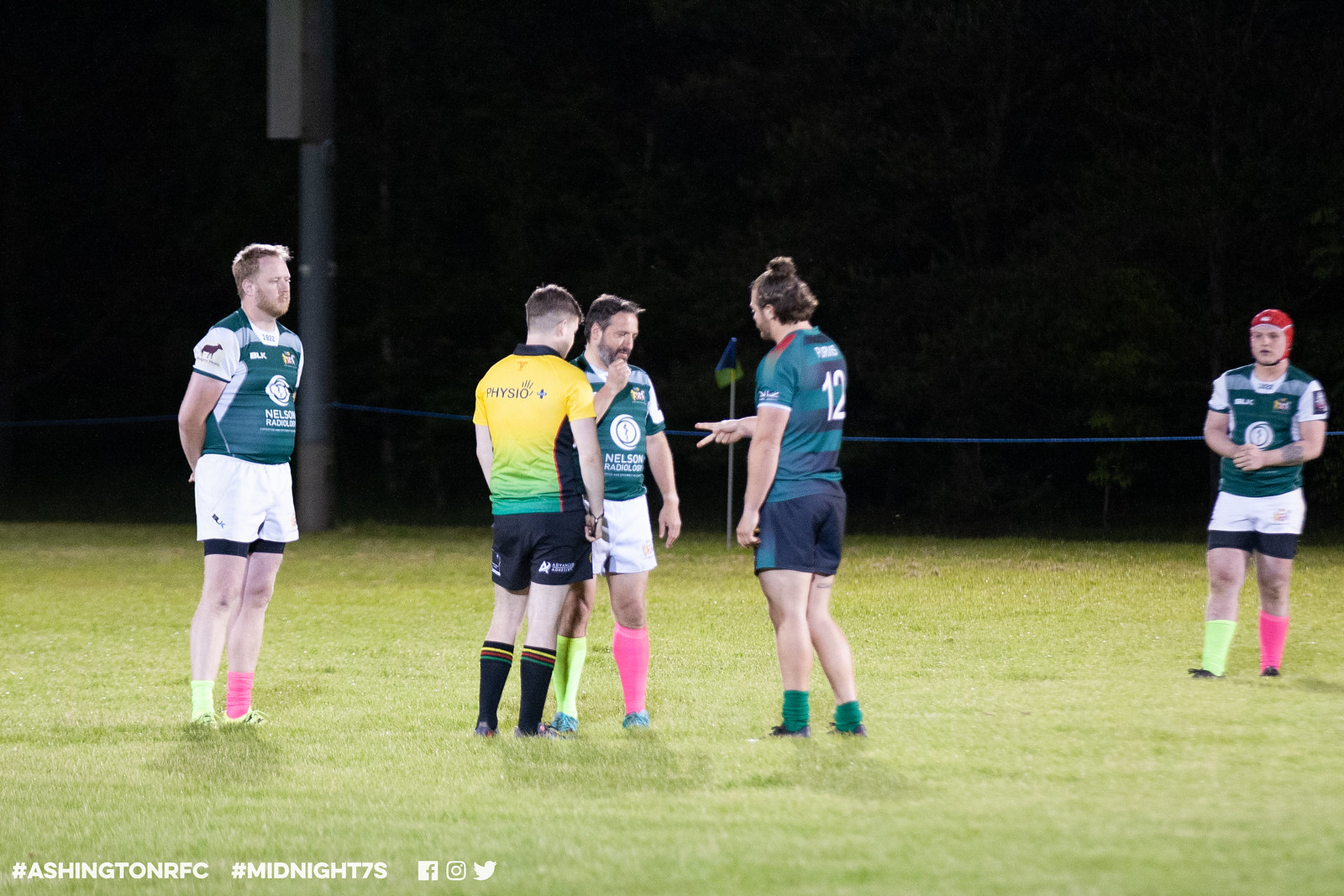The rectangular image captures a nighttime soccer scene on a field. At least five players are visible, each dressed in varied jerseys and shorts, though none seem to be wearing much equipment like shin pads. The scene is brightly lit by artificial lighting from above, casting stark illumination on the players against a predominantly dark background. Three players are donning green jerseys with white shoulders and white shorts, sporting mismatched socks: one in lime green and the other in pink. Notably, their socks are worn at different lengths—some pulled up while others are scrunched down around their ankles.

Another player, presumably an opponent, is clad in a green-and-blue striped jersey paired with dark shorts and black socks featuring yellow, red, and green accents. A figure who appears to be the referee stands in a bright yellow jersey and black shorts. The focal point of the photograph is the interaction - the two central players, one with a raised fist and the other holding out two fingers in a scissors motion, seemingly engaged in a game of rock-paper-scissors, while the referee looms over them and others watch.

In the backdrop, a blue rope demarcates the field area, and one can discern a pole, a fence, and faint outlines of trees. The bottom left corner of the photograph features white text with the hashtags #AshingtonRFC and #MidnightS7S alongside the logos for Facebook, Twitter, and Snapchat.